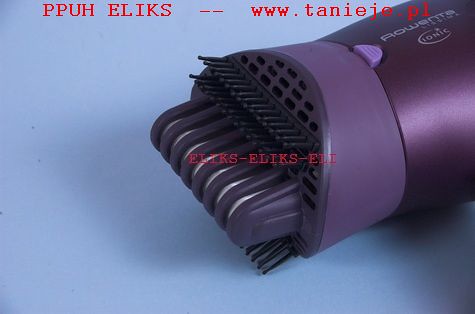The landscape-oriented image depicts an electric personal grooming device, likely used for depilation or haircuts, featuring a purplish-pink and burgundy design with matte black accents. The device, positioned from the top right towards the center, appears to be a shaver with protruding bristles and possible blades in plastic safety casings. Prominently displayed are some red and white text, including "P-P-U-H-E-L-I-K-S" and "Rowetta Ionic," as well as a Polish web address, "www.taniejo.pl." The background is a mix of bluish and gray hues, with the central part of the image showcasing the letters "L-X-L-X-L-E" in thin red font. The overall appearance suggests a sophisticated, complex grooming tool, though its specific function remains ambiguous.